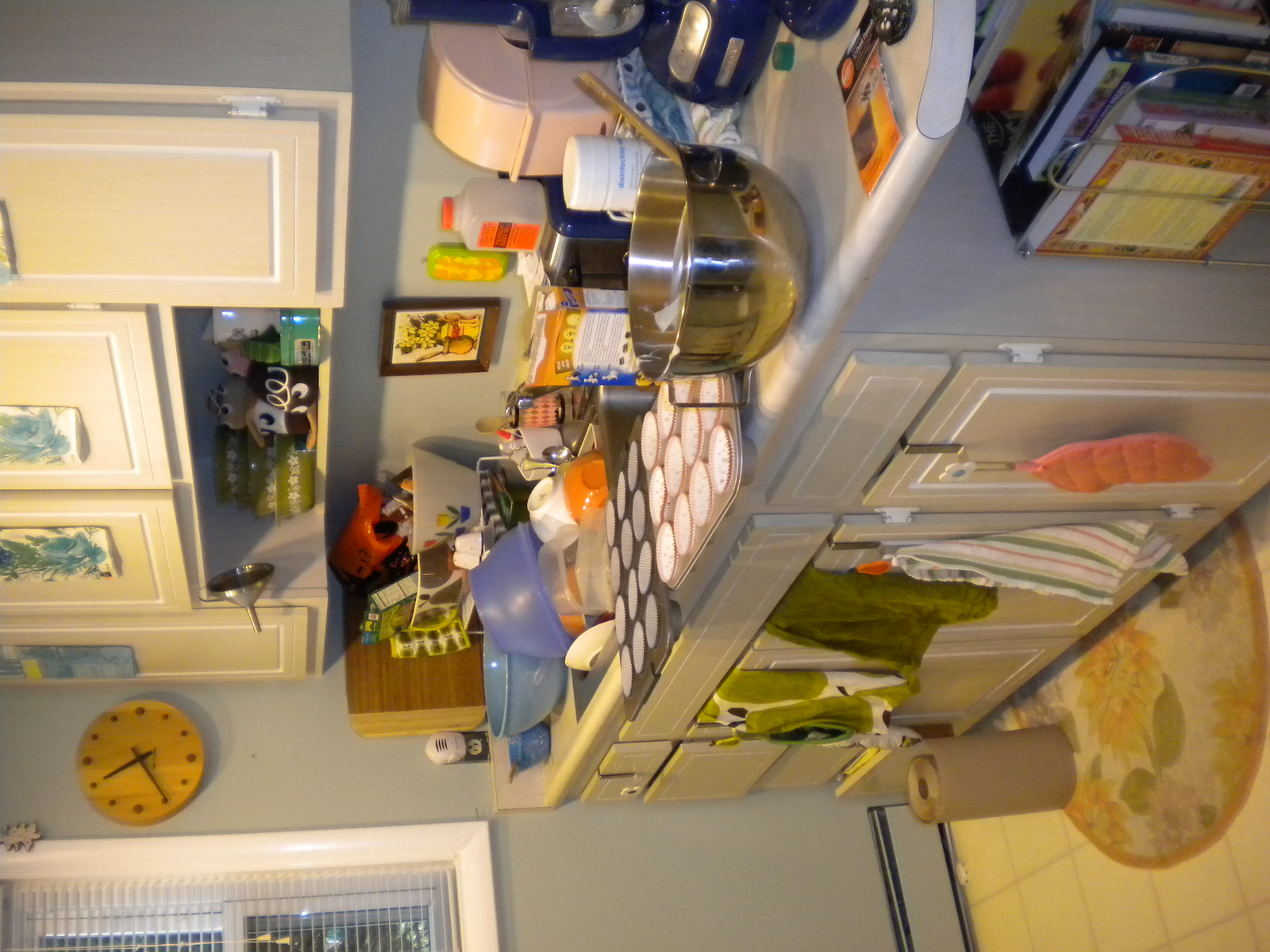This photograph showcases a kitchen interior that has been rotated 90 degrees counterclockwise, presenting the scene sideways. The kitchen counter features a sleek grey surface, while the lower cabinets and drawers are painted a beige eggshell white, complemented by white frames. The hardware on these cabinets is indeterminate, but there are metal hooks attached, reminiscent of dollar store finds, holding dish towels and pot holders.

The countertop itself is cluttered with an array of cooking items, including chrome mixing bowls, blue plastic bowls, and various baking trays. The backsplash is a light grey or blue, adding a subtle contrast to the overall decor.

The upper cabinets share the same eggshell white coloring with white frames, continuing the cohesive design. The countertop and nearby areas are packed with utensils, products, and packaging, making the space appear very busy.

On the left wall, a wooden circular clock with black hands and dot markers instead of numbers hangs prominently. Part of a window with a white frame and white blinds is also visible. The floor is covered with beige off-yellow tiles, reminiscent of 90s decor, and a faded circular rug with a floral pattern lies partially underneath the counter area, indicating where one might stand while cooking. An additional detail is the roll of brown paper towels resting on the floor. Scattered around the scene are various bowls and mugs in different colors, including orange and white, contributing to the overall impression of a well-used, lived-in kitchen seen from an unusual perspective.